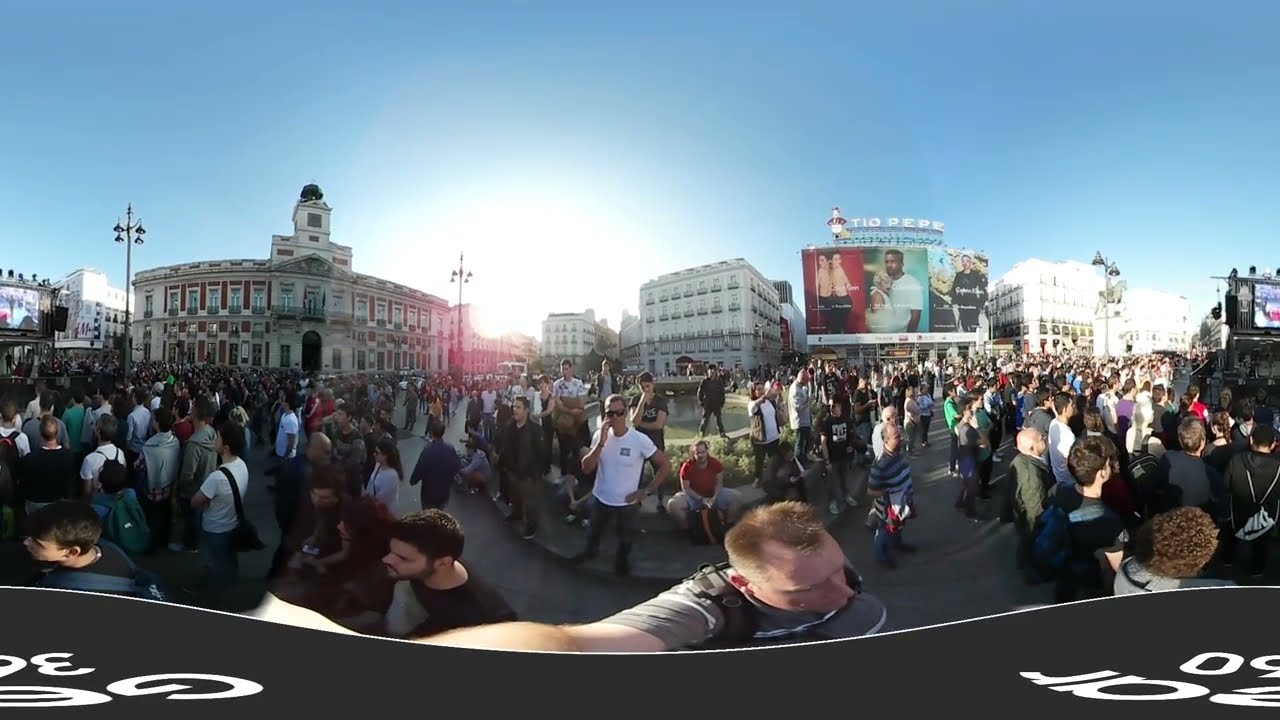This image is a wide-angle, panoramic shot capturing a bustling plaza on a bright, early day, possibly in a European city. The foreground of the image features a man with short hair, wearing a gray shirt and possibly something over his right shoulder, holding a camera, perhaps with a selfie stick, as he takes the photo. His extended arm, slightly distorted, almost reaches the left side of the image. Behind him, a diverse crowd fills the plaza, standing and sitting around various focal points.

On the left, there's a prominent two-story building with a rounded side and architectural details including light poles, a base supporting another section topped with a small dome. Interspersed among the crowd in front of this building are more people, enhancing the scene's liveliness. To the immediate right of this building is another segment of the image showcasing people in a grassy area centered around a circular feature, possibly a fountain. 

The middle part of the panorama is notably distorted, affecting the clarity of the people depicted there. Beyond this, a street can be seen, lined with people on both sides and leading up to a large billboard featuring a white sign, unreadable in this context.

Further to the right, the image continues to show more buildings—one resembling an office building—with additional people in the foreground. The sky is a radiant blue with the sun glowing from behind the buildings, casting bright light and shadows.

At the very bottom, near the man's outstretched arm, is a white line that underscores the series of images, dipping slightly in the middle, possibly indicating where the images join. Beneath this line, a gray background with white lettering can be seen in the lower corners. The overall scene conveys a dynamic urban environment teeming with activity and architectural diversity.